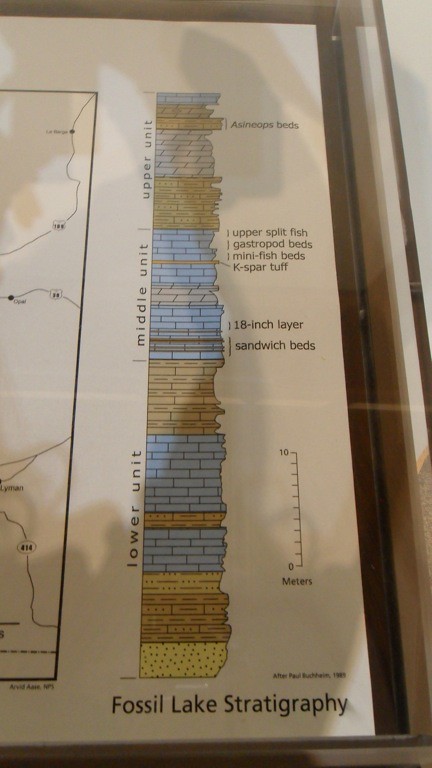This image appears to be a detailed graphic encased within a brown frame, likely observed in a museum or a natural history exhibit, as suggested by the reflections and shadows on the glass. The centerpiece of the graphic is an illustrative cross-section that vividly depicts the stratigraphy of Fossil Lake. The stratigraphy is meticulously illustrated in various colors, including shades of yellow, brown, and light blue, representing approximately 15 different sedimentary layers.

On the right side of the graphic, there's descriptive text, including a label noting an "18 inch layer sandwich beds," accompanied by a scale bar marked in increments from 0 to 10 meters, providing a sense of the layers' actual size. This scale allows viewers to appreciate the depth and compaction of the sediment over time. At the bottom of the illustration, the title "Fossil Lake Stratigraphy" is clearly printed in bold black letters, indicating the geological focus of the display. This visual and textual information seems dedicated to explaining the formation and composition of the lake's sedimentary layers, effectively educating viewers on the geological history preserved within the layers of rock.